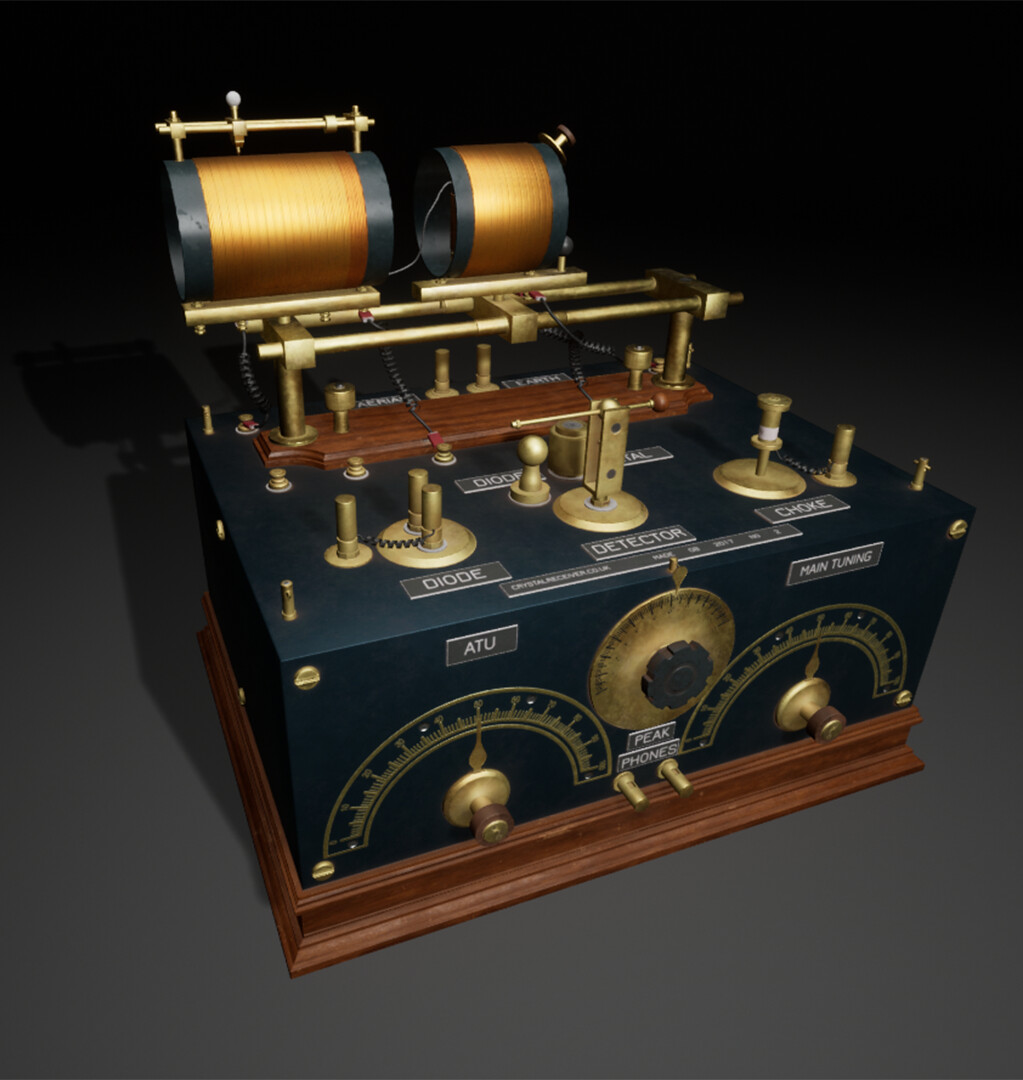The image depicts a 3D rendering of vintage audio equipment, resembling an early radio. The device features a reddish-brown wooden baseboard supporting a black rectangular prism. Prominently, the front of the prism displays two half-moon scales with central golden dials, labeled "ATU" and "Main Tuning" respectively on silver nameplates above them. Between these scales, a large central gold dial with a black cog is labeled "Peak" and "Phones," with two golden switches beneath the labels. 

On top of the black box, numerous vertical golden rods are arranged: a left-hand group labeled "Diode," a central section featuring a gold fork-shaped object with a horizontal golden dowel capped by a red ball indicated as "Detector," and a right-hand group labeled "Choke." At the rear, a wooden section sits atop the box, flanked by two golden supports connected by horizontal golden rods. Additionally, the left side features two horizontal black hollow cylinders adorned with gold lines.

The background showcases a gradient transitioning from dark gray at the bottom to black at the top, adding depth and contrast to the image. The intricate detailing and combination of black, gold, and reddish-brown elements lend the object an authentic, historical appearance reminiscent of early radio equipment.